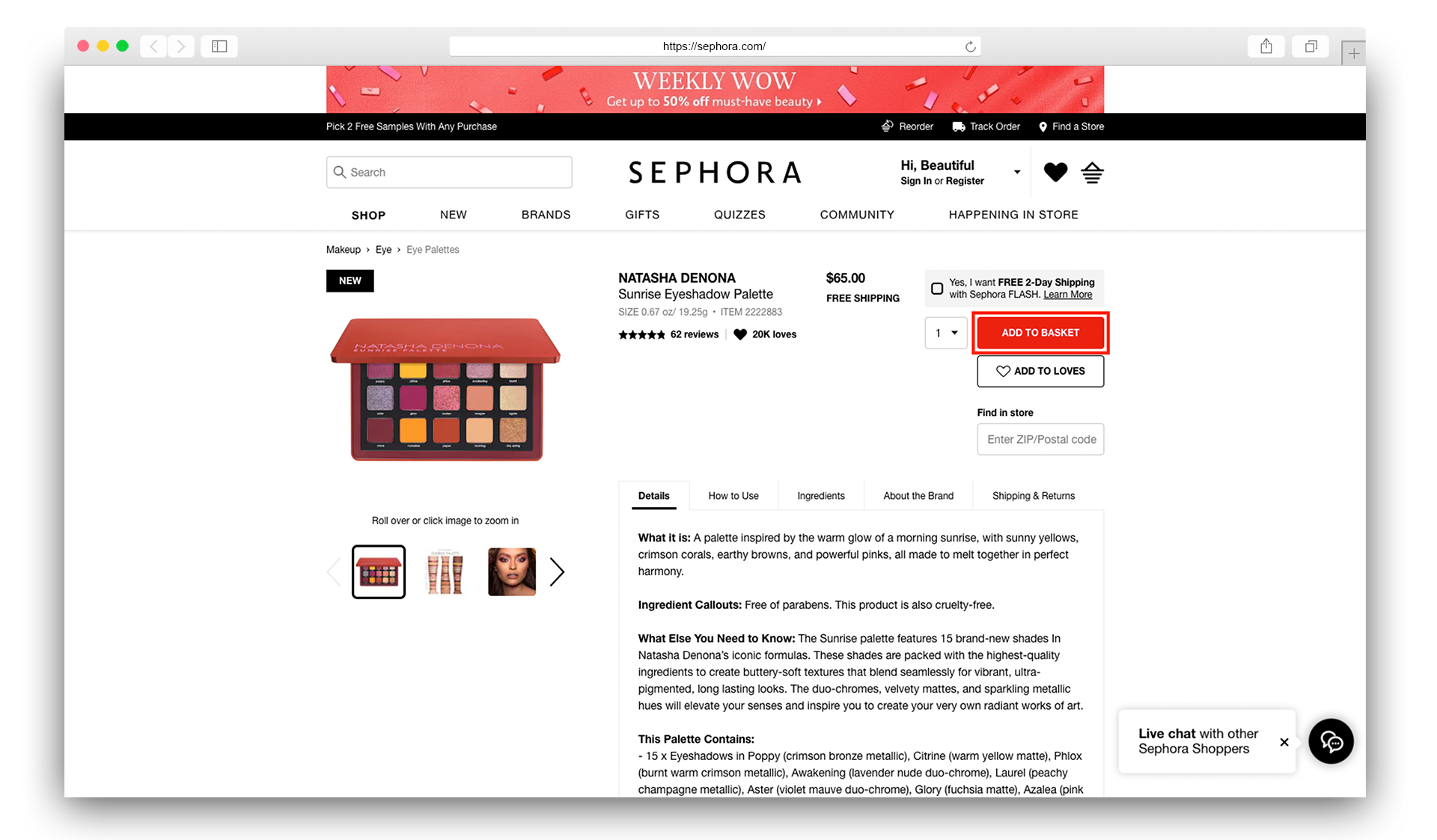This screenshot captures a section of the Sephora support website. At the top, there is a prominent advertisement for the "Weekly Wow," offering up to 50% off on must-have beauty products. The ad features a pink-to-red gradient background adorned with images of various lipsticks and beauty items.

Directly below the advertisement, there is a black bar announcing that customers can "Pick Two Free Samples" with any purchase. This bar is followed by three menu options: "Track Order," "Find a Store," and a white search bar. 

Centered on the page is the iconic Sephora logo, alongside a friendly greeting, "Hi Beautiful," with options for users to "Sign In" or "Register" for an account. Below this, visitors can navigate through several menu options such as "Shop," "New," "Brands," "Gifts," "Quizzes," "Community," and "Happening in Store," with the current focus on the "Shop" section.

In this section, the featured item is the Natasha Denona Sunrise Eyeshadow Palette, priced at $65. This palette draws inspiration from the warm hues of the morning sunrise, featuring a harmonious blend of sunny yellows, crimson corals, earthy browns, and vibrant pinks. The eyeshadow palette boasts 15 brand-new shades and highlights its cruelty-free formula. 

Additionally, there is a "Live Chat" support button located in the bottom right corner of the screen, offering immediate assistance to customers.